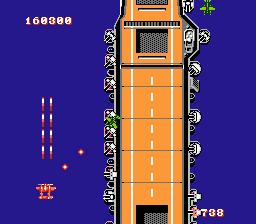The image is a screenshot from an unspecified video game, featuring a vertical, orange-tinted path resembling a road or a battleship deck, with white dashed lines running down its center and white pinstriping along the edges. The background is a vivid blue, enhancing the clarity of the scene. In the top left corner, the player's score is prominently displayed as 160,300, while additional score markers of 738 are visible in both the top right and bottom right corners.

Amidst the action, several airplanes are seen firing missiles towards the left side of the image, where cannons on the orange structure seem to retaliate with orange-hued rockets. A small, orange robot-like figure is also present, emitting red and yellow projectiles toward the road-like structure. The right side of the image features a green airplane contributing to the chaotic aerial battle. The road is notably edged with gray and contains sporadic gray squares, adding to the game's intricate details. Red lines, possibly indicating life graphs, are also visible, contributing to the overall dynamic and visually complex scene.